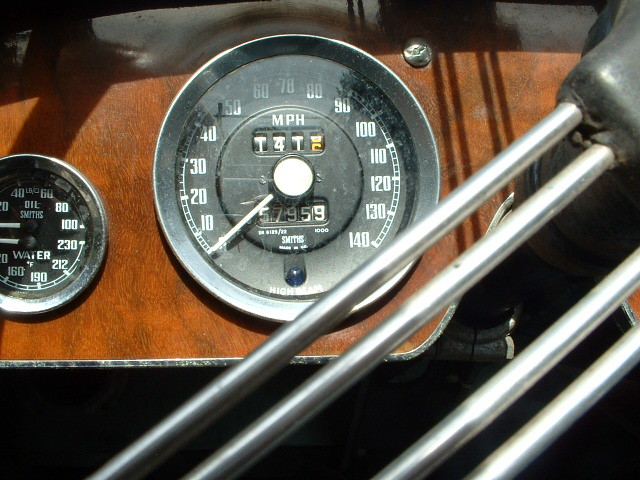The image displays two spherical dials that appear to be part of a vehicle's dashboard or an industrial control panel. Dominating the center of the frame is a large gauge with a highly reflective, glass-covered face. This gauge features a pristine black background with stark white lettering. The dominant display indicates speed in miles per hour (MPH), with numbers ranging from 0 to 140 in increments of 10. The needle, currently pointing to zero, pivots from a central hub, and just below this hub is an odometer reading "57959."

To the left of the primary speedometer is a smaller, similarly spherical gauge, also ensconced in reflective glass. This secondary dial appears to monitor pressure or temperature, with its measurements scaling up to 230 before dropping back down to 212, indicating a cyclical or dual-function range. White lettering labels the top of this smaller gauge with "Oil" and the bottom with "Water," signifying its dual-purpose monitoring capability. Both dials are framed by sleek silver bars running through the image, adding a touch of industrial elegance.